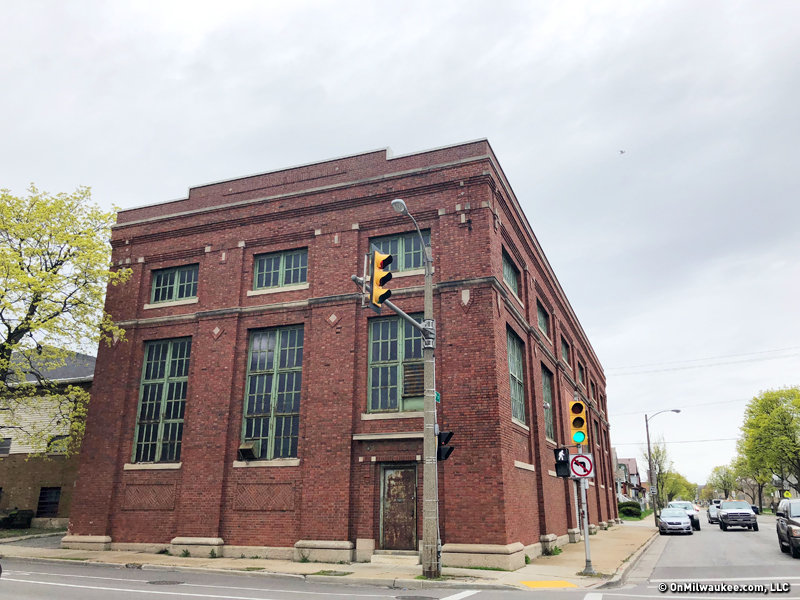This image captures a bustling street intersection dominated by a weathered, deep red brick building on the left-hand side. This old structure, possibly out of service, features a rusty metal door stripped to its original wood color and two rows of windows—a lower row with long windows spanning two stories and an upper row of smaller ones. Adjacent to the building stands a green tree with light leaves, while the sidewalk of cement snakes through the foreground. The right side of the image reveals a street scene with multiple cars facing the camera, a green traffic light, streetlights, and a pedestrian crosswalk flashing the walking man symbol. Cloud-filled skies add an overcast blue hue to the setting, with additional green trees dotting the background. The bottom of the image displays the text "copyright milwaukee.com LSC" in white.